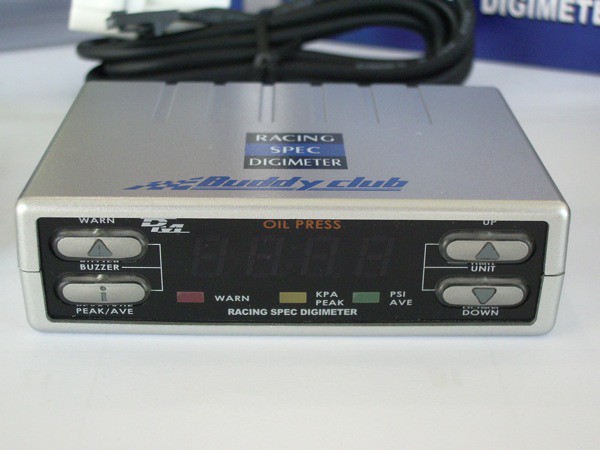In the image, we see a piece of electronic equipment named the "Racing Spec Digimeter" by Buddy Club, presumably used in racing scenarios. The device features several controls and indicators. Prominently displayed are two buttons labeled "Down" and "Up," accompanied by a smaller arrow pointing to the word "Unit." There is a small red light labeled "Warn" which is currently off. Adjacent to this light, there is an indicator marked "KPA Peak" beside a non-illuminated yellow light, and nearby is another green light labeled "PSI AVE," also not lit. 

Below these indicators, the device bears the label "Racing Spec Digimeter" again. On the left side, there's a "Peak/AVE" button with an upside-down exclamation point symbol. Above this button is one marked with a triangle and exclamation point, labeled "Buzzer." Above it, another "Warn" label is present, and the designation "DM" can be seen. 

In red letters, the display reads "Oil Press," but there are no active LED digits visible. The device is connected to what looks like a black plug at the back. This entire setup is placed on a white table, with daylight streaming in from the background. A grayish-white surface visible could be either the table or the floor, and "Digimeter" can be partly seen in the background. A dark blue surface is also visible, adding to the contrasting colors in the image.